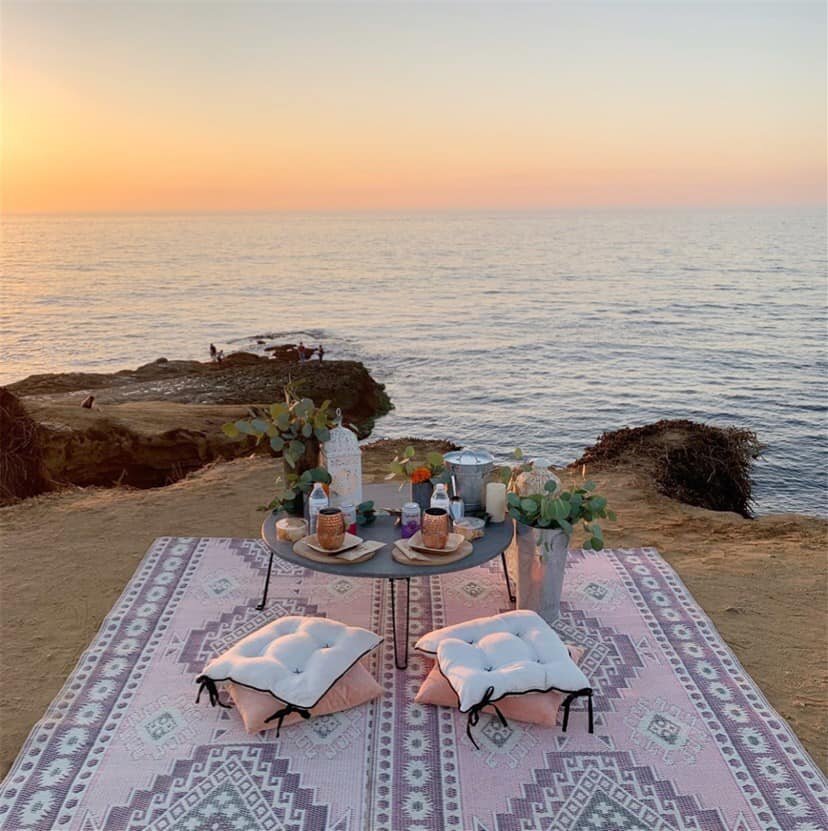This image showcases a picturesque and ornate picnic set up on a coastal dirt area that leads right into the expansive ocean. The vibrant sky, painted in hues of orange, yellow, and pink, suggests the sun is either rising or setting, casting a serene glow over the scene. The sprawling sea, dotted with calm waters, extends to the horizon, with a small rock formation jutting slightly into the ocean and a few visible people near the water's edge.

In the foreground, a lavish picnic setup features a patterned carpet in shades of gray and light pink, laid delicately over the dirt. Atop this carpet rests a gray circular table accompanied by a silver vase filled with a flower arrangement, an ice bucket, a candle holder, and various cups, glasses, and plates. Plush pillows in white, pink, and gray are arranged around the settings, offering a cozy seating area. The overall atmosphere is one of tranquility and elegance, accentuated by the beautiful interplay of natural colors and curated picnic elements.